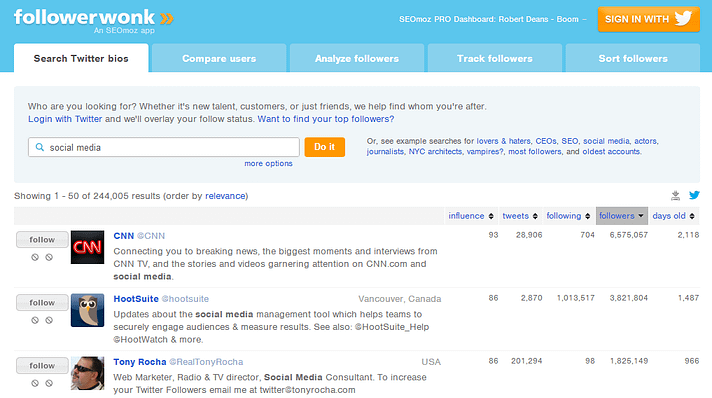Title: Detailed Overview of “Follower Wonk” Website

Description:
The image showcases an introduction to a website named "Follower Wonk," prominently displayed in the upper right-hand corner. The site offers the option to sign in with Twitter through an orange button, conveniently located in this section. 

Central to the webpage, slightly toward the right, there are mentions of "S-E-O-N-O-Z" and "Pro Dashboard,” suggesting the presence of tools oriented towards professional SEO management. The name "Robert Deans" is also visible in this area, potentially referencing a user or a key feature on the interface.

Follower Wonk describes itself as an SEO-centric application designed for detailed Twitter analysis. The platform boasts features such as the ability to search Twitter bios, compare users, analyze and track followers, and sort them accordingly. It seems to cater to individuals or businesses aiming to manage social media accounts effectively, particularly those with a significant follower base.

Additionally, the website promotes its utility in finding new talent, customers, or friends by leveraging Twitter data. The tagline suggests, "Who are you looking for? Whether it's new talent, customers, or just friends, we help find whom you're after." This indicates a comprehensive focus on enhancing social media engagement and follower insights. 

A prominent call to action encourages users to log in with Twitter, promising to overlay the user's follow status for a more integrated and personalized experience. The site further entices potential users with a question: "Want to find your top followers?" indicating a specialized feature for identifying key followers.

Overall, Follower Wonk appears to be a robust tool aimed at optimizing social media strategy through in-depth follower analysis and engagement management.